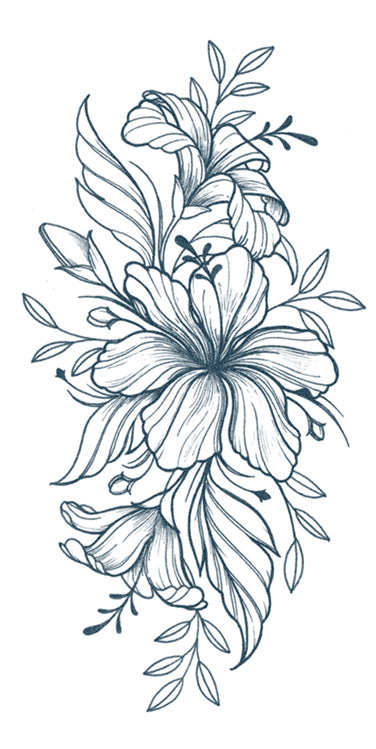The image displays a detailed drawing of a flower bouquet, rendered in either dark blue or black ink on a plain white background. Central to the composition is a large, symmetrical flower with six petals, its center adorned with a small stem holding five tiny petals. Flanking this primary bloom are additional flowers and leaves, intricately arranged upwards and downwards along the central vertical stem. The bouquet includes three prominent blooming flowers, each extending leaves from their stems, creating a visually balanced and harmonious pattern. The artwork is distinguished by its fine lines, emphasizing the meticulous use of a black pen or blue marker to capture every detail.